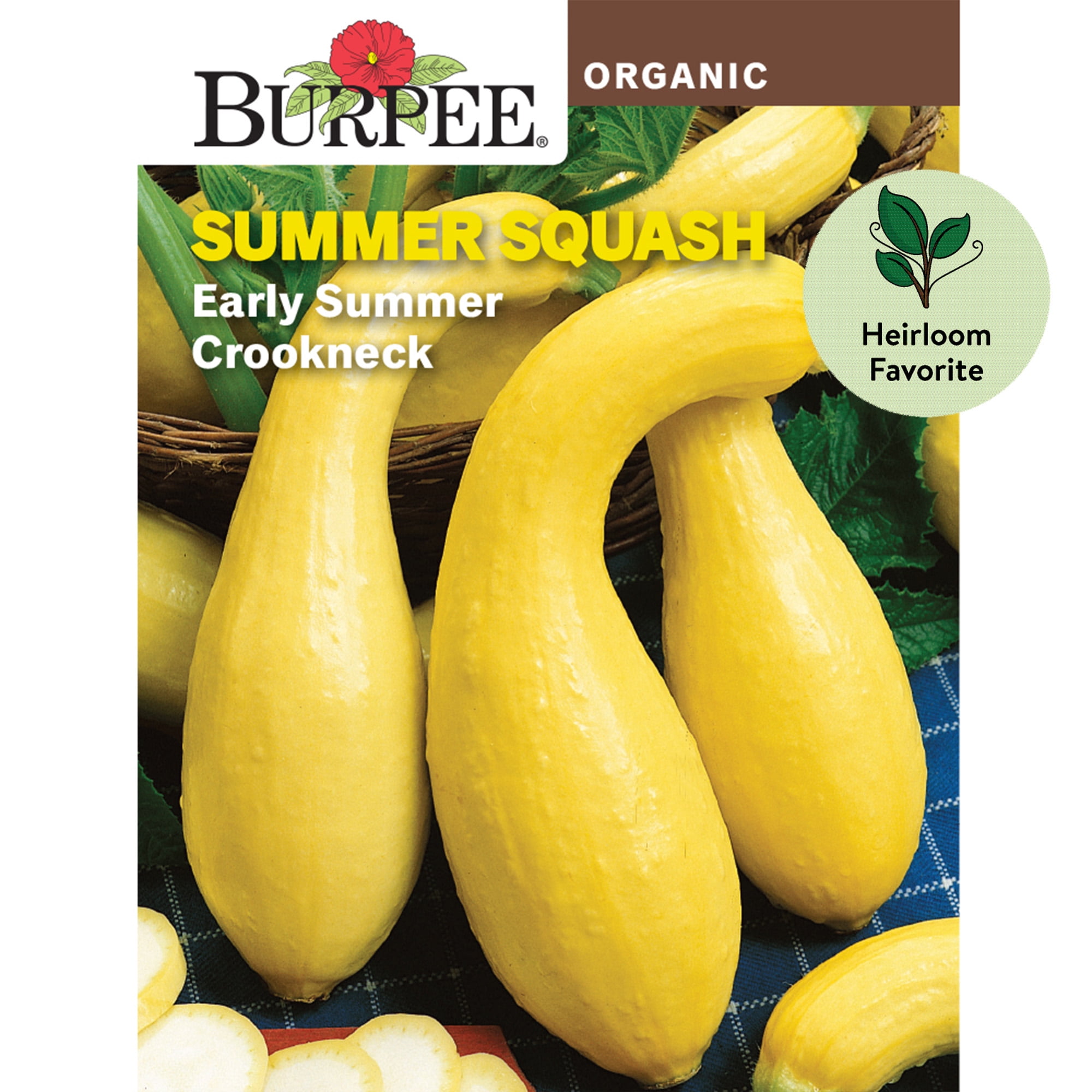This vertically aligned rectangular image appears to be the front of a large seed packet from the Burpee brand. In the upper left corner, "BURPEE" is prominently displayed in all caps with black letters against a white background. Behind the R, N, and P in "BURPEE," there is a depiction of a red flower with a yellow center and green leaves. Adjacent to this, in the upper right corner, "ORGANIC" is printed in white, all-caps letters on a brown rectangle. Underneath "BURPEE," the text "SUMMER SQUASH" is featured in bold yellow, all caps. Below that, "EARLY SUMMER CROOKNECK" is written in white. Along the right edge of the packet is a small circular emblem with a light green background, featuring an image of some plants and labeled "HEIRLOOM FAVORITE" in black text. The main background is vibrant and colorful, showcasing three large vertically-aligned yellow squashes surrounded by green leaves. Additional squashes are visible lying down in the lower right corner and several sliced pieces are depicted in the lower left corner. In the distant background, there is a faint image of what appears to be a bucket with other vegetables or leaves, potentially okra.